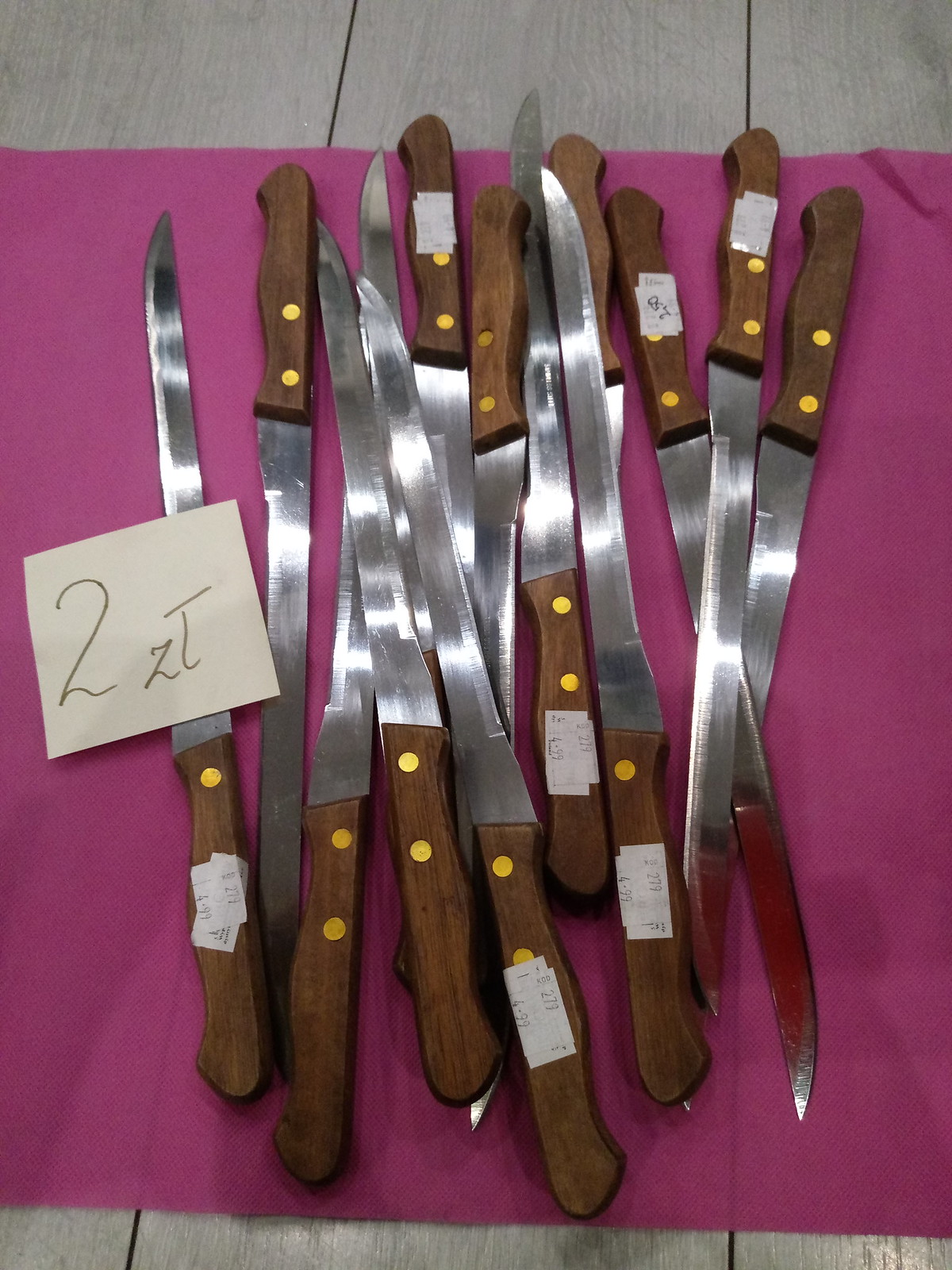This digital photograph, with indistinguishable indoor or outdoor setting, features a light gray wooden surface composed of three planks separated by thin black strips. Central to the image is a large purple square piece of construction paper. Arranged on this paper are approximately fifteen identical knives, characterized by their long, thin silver blades and dark brown wooden handles, each affixed with two lighter-colored spots where the blade attaches. The knives are laid out in various orientations, with some handles pointing up and others down. Notably, a light blue sticky note marked with "2ZT" in gray pencil is affixed to the knife on the far left. Additionally, several handles bear white price stickers, and one sticker near the top reads "$2.50", suggesting they are being sold at this price.